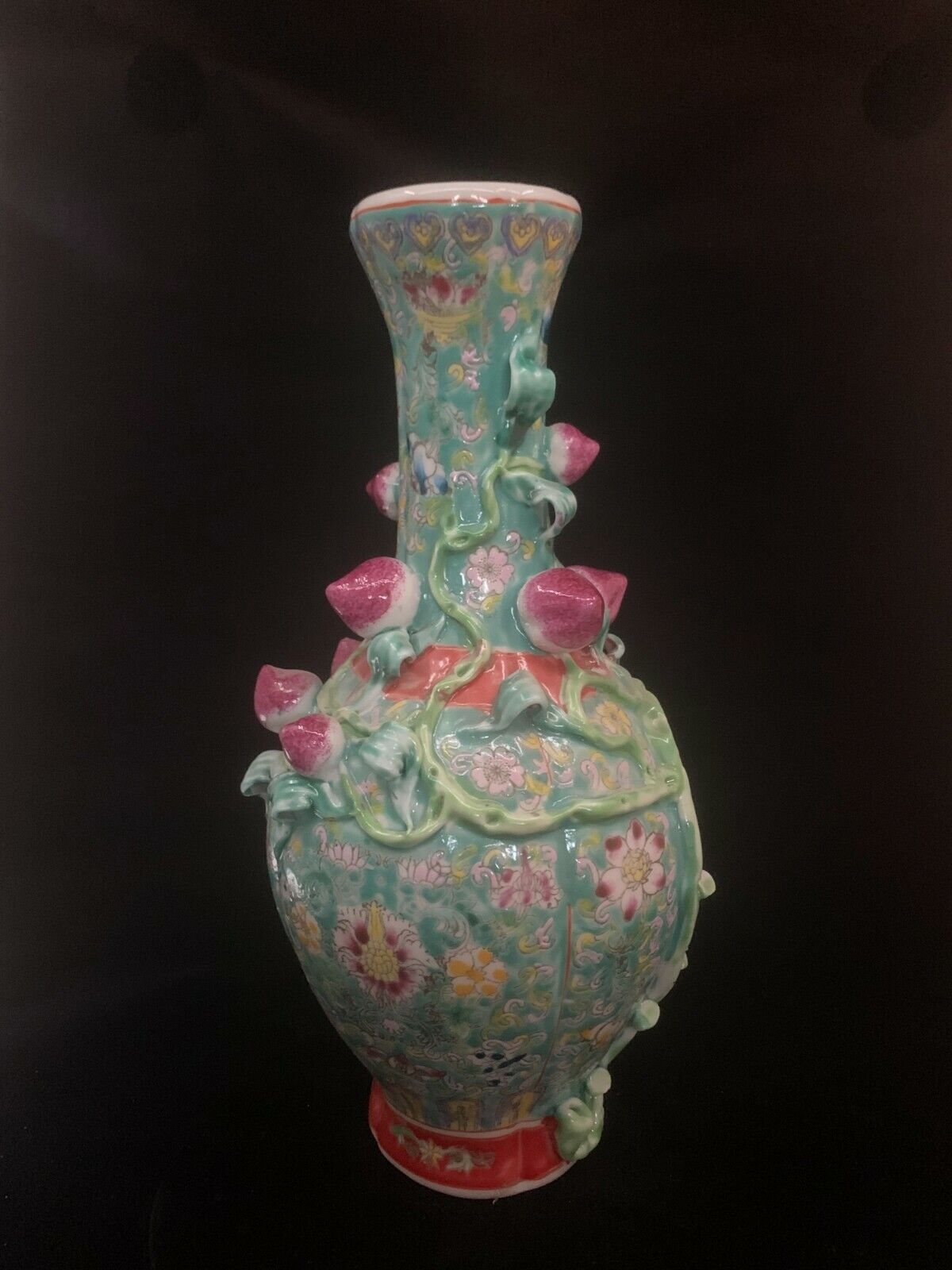This photograph depicts an urn-shaped antique vase, potentially with oriental origins from an Asian country such as China or India. The vase's primary jade green color is accentuated with intricate filigree work resembling climbing vines or ivy. These raised sculptural designs showcase natural motifs, including strawberries, leaves, and various flowers. The vase features detailed inlaid flowers of assorted colors, including maroon, white, and orange, with fine red circular paintings accentuating the base and neck. Yellow heart shapes outlined in blue add to its elaborate decoration towards the top. The vase narrows at the neck, expands in a rounded form, and then tapers back to a small, orange pedestal base adorned with further floral designs. The design work adds to the overall aesthetic, hinting at elements like dragons or additional flora at the very bottom.